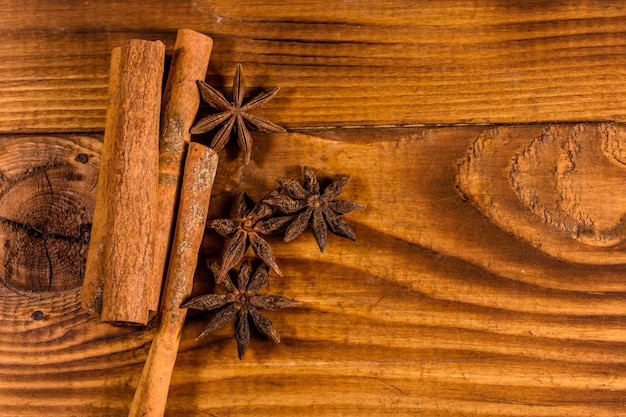This image is a rectangular, bird's-eye view close-up of a stained wooden surface, wider than it is tall. The background surface, likely pine with a wide grain, has been stained a dark chestnut brown, exhibiting a honey color. You can appreciate the textures and natural accents in the wood, such as the visible grooves and knot holes, which suggest an old, dry, and rough finish. On the left side of the image, there are four cinnamon sticks, varying in thickness, with a similarly dry and rough texture to the wood underneath. Towards the center right of the image, there are four star anise pods. These dark brown star anises each feature six or seven tendrils radiating from a central point and appear quite dry, similar to how they would look if left exposed to the air for a long time. The overall composition highlights the natural, rustic attributes of both the wooden surface and the dried spices.